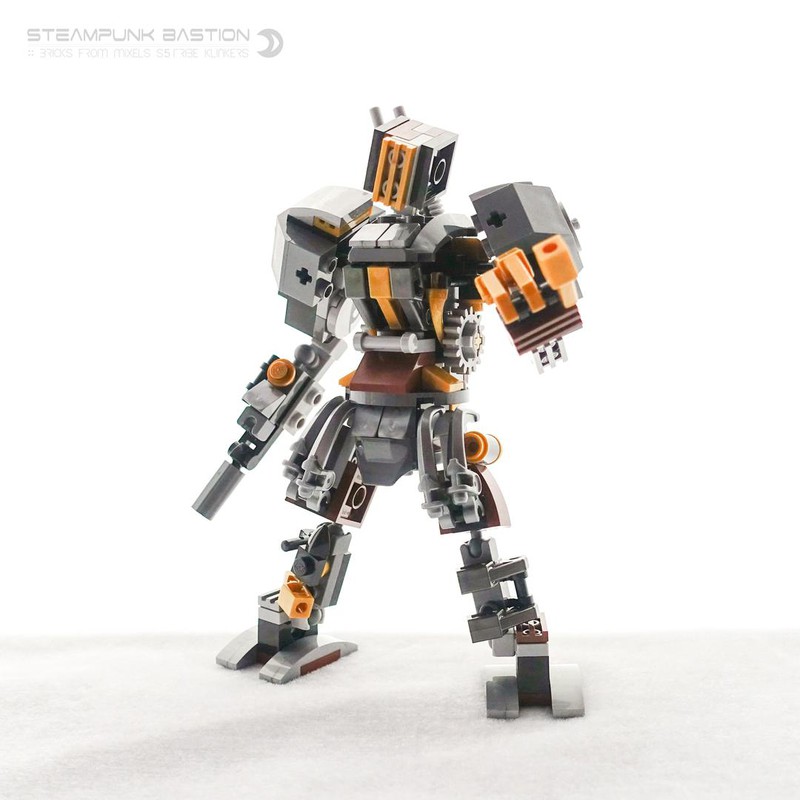The image depicts a detailed, humanoid robot seemingly constructed from Lego components, embodying a robust steampunk aesthetic as indicated by the text “Steampunk Bastion” in the top left corner, accompanied by a partially legible subtext and a distinctive logo resembling a reversed crescent moon. The robot stands prominently against a white background, displaying a dynamic pose with legs apart and one arm raised, suggesting readiness for combat. The figure is composed of various interlocking pieces with a predominant color scheme of gray and orange, accented by touches of brown and red at certain joints and surfaces. The robot's head, featuring an orange-blocked front with three vertical lines, is a clear focal point. It has broad shoulders, a slightly tilted head, and in its right hand, it brandishes a small Lego gun. Additionally, a gear is visible on the left side of its waist, which likely facilitates twisting motions. The left hand of the robot is distinctive with three orange fingers, further contributing to its mechanical, yet anthropomorphic design.